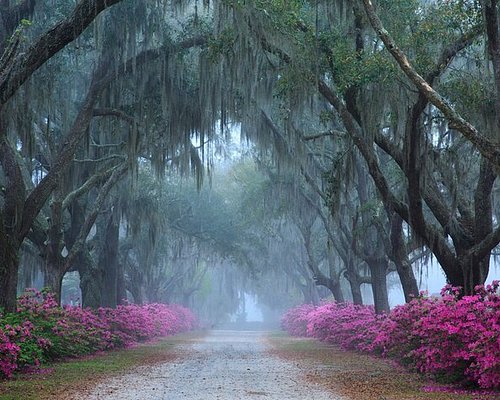This photo depicts a serene, moody scene of a grey gravel pathway meandering into the misty distance, flanked by two rows of large trees. The trees, which have moss and various elements hanging down, create a canopy over the road, adding to the atmospheric depth of the setting. At the base of these trees are numerous bushes bursting with vivid pink and purplish flowers, providing a striking contrast to the otherwise muted, foggy environment. The gravel path itself is bordered by patches of brown dirt and encroaching green grass, contributing to the natural, untouched feel of the landscape. The overall tone is one of gentle melancholy, reminiscent of a scene from Forrest Gump, with the mist and blue hues enhancing the dreamy, rainy ambiance.